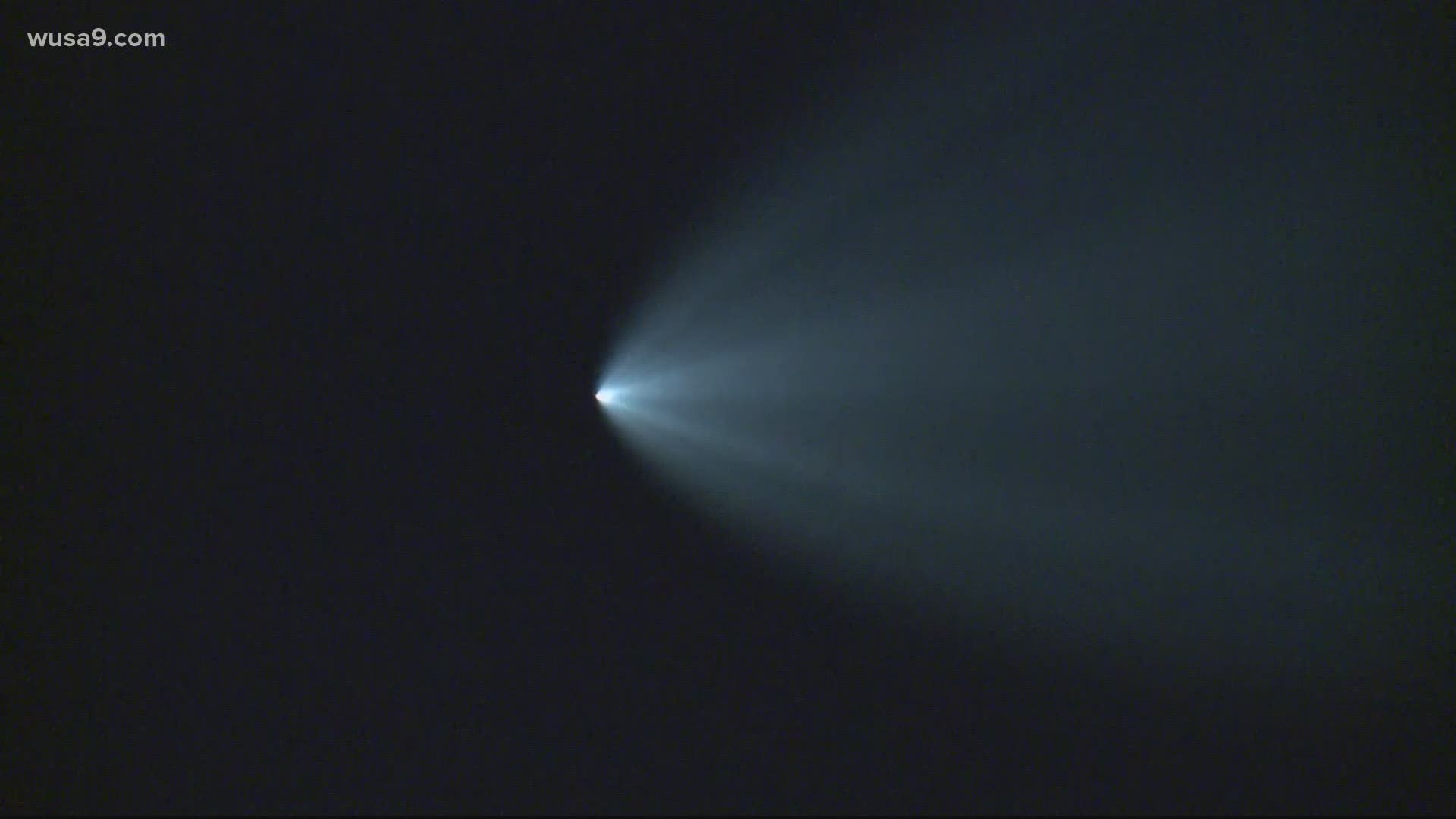The image features a predominantly black background with a striking beam of light in the center, resembling a flashlight piercing through the darkness. The focal point is a bright circular dot of white light situated almost dead center, from which a parabolic beam of light radiates outward. This beam, which forms a shape reminiscent of a C if made with your left hand, extends from the bright center to the right edge of the image, gradually dissipating into the darkness. The light creates a gradient effect with grayish rays illuminating the surrounding blackness. The composition is horizontal, almost like a landscape, and in the upper left corner, a watermark reads WUSA9.com.